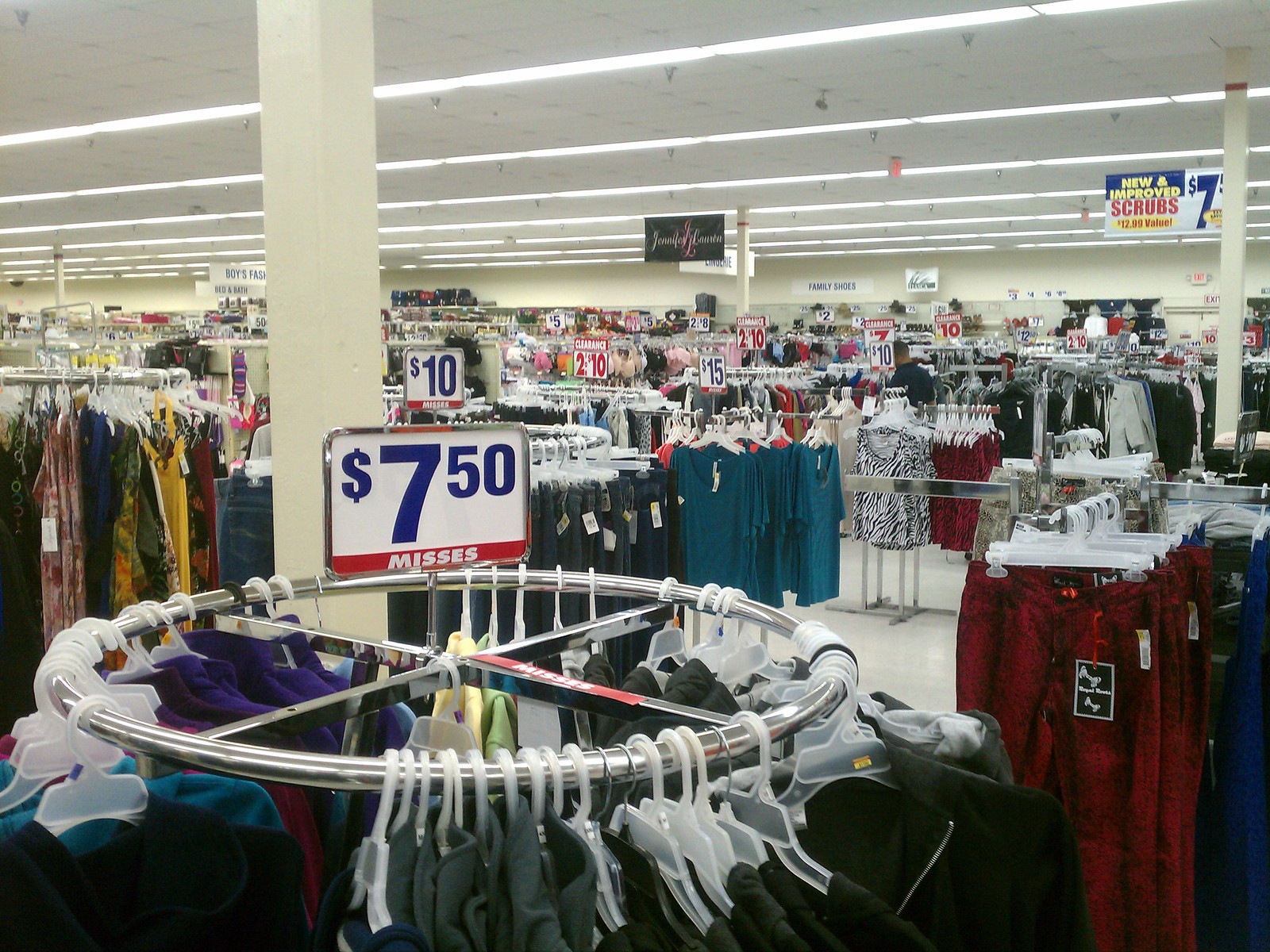The photograph captures an interior view of a large department store, potentially a Walmart, characterized by its vast array of merchandise and organized layout. In the bottom left corner, there is a circular clothing rack filled with an assortment of colorful shirts in hues of blue and purple, all neatly hung on white plastic coat hangers. This rack is topped with a rectangular sign that prominently displays a price of $7.50 in purple text on a white background.

The store extends into the background, revealing additional sections with blue shirts and possibly red pants, all displayed on similar circular racks. A stark white post is seen on the left side, extending from the floor to the ceiling, contributing to the store's bright and clean aesthetic dominated by white walls and ceiling.

A notable feature on the top right of the image is a sign labeled "Scrubs," indicating a dedicated section for medical apparel. Ceiling lights illuminate the entire space, ensuring a well-lit shopping environment. In the center of the image, another price sign, marked $10, is visible, further emphasizing the store's budget-friendly offerings. The absence of shoppers in the photo lends a serene, uncrowded feel to the otherwise bustling retail setting.